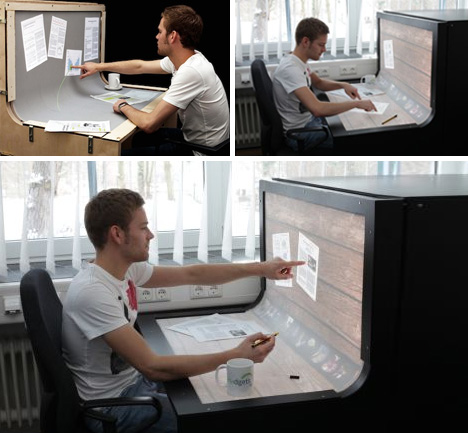In this photograph, a young Caucasian man with brown hair, dressed in a white shirt adorned with red and black designs, is working at a modern, gray-surfaced desk that appears to be made of a 3D-looking material, possibly wood. He is seated on a black chair and is consistently seen pointing at various documents on the desk and on the wall. A white mug sits on the right side of his desk. Surrounding him are multiple pieces of paper scattered across the desk and attached to the wall, where he directs his attention. On his left wrist, he wears a watch. Natural light streams in through a window visible in the background, illuminating the workspace. The windows' sturdy structure and the gray-colored walls enhance the scene's ambience. The man also holds a pencil in his right hand, actively engaging with the materials laid out in front of him.